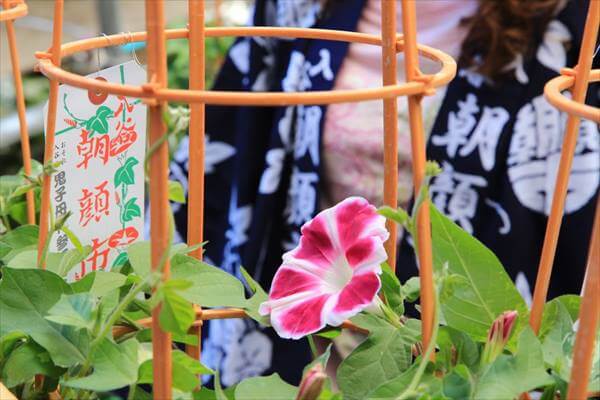This close-up color photo captures a detailed scene in a garden, predominantly showcasing bright orange, circular tomato cages made of metal. The cages, painted in bold orange to possibly prevent rust, are designed to support growing tomato plants. Prominently, one cage features a hanging tag with Japanese or Chinese characters and an illustration of tomatoes on the vine, suggesting it offers installation instructions.

In the foreground, vibrant green foliage surrounds a singular, delicate petunia with striking maroon and white petals. This flower, nestled within one of the orange cages, adds an elegant touch to the image. Behind the main subjects, slightly out of focus, hang blue tapestries adorned with white characters, likely Japanese or Chinese calligraphy, adding an additional cultural layer to the scene. The overall composition is both colorful and serene, blending elements of nature and subtle human influences.